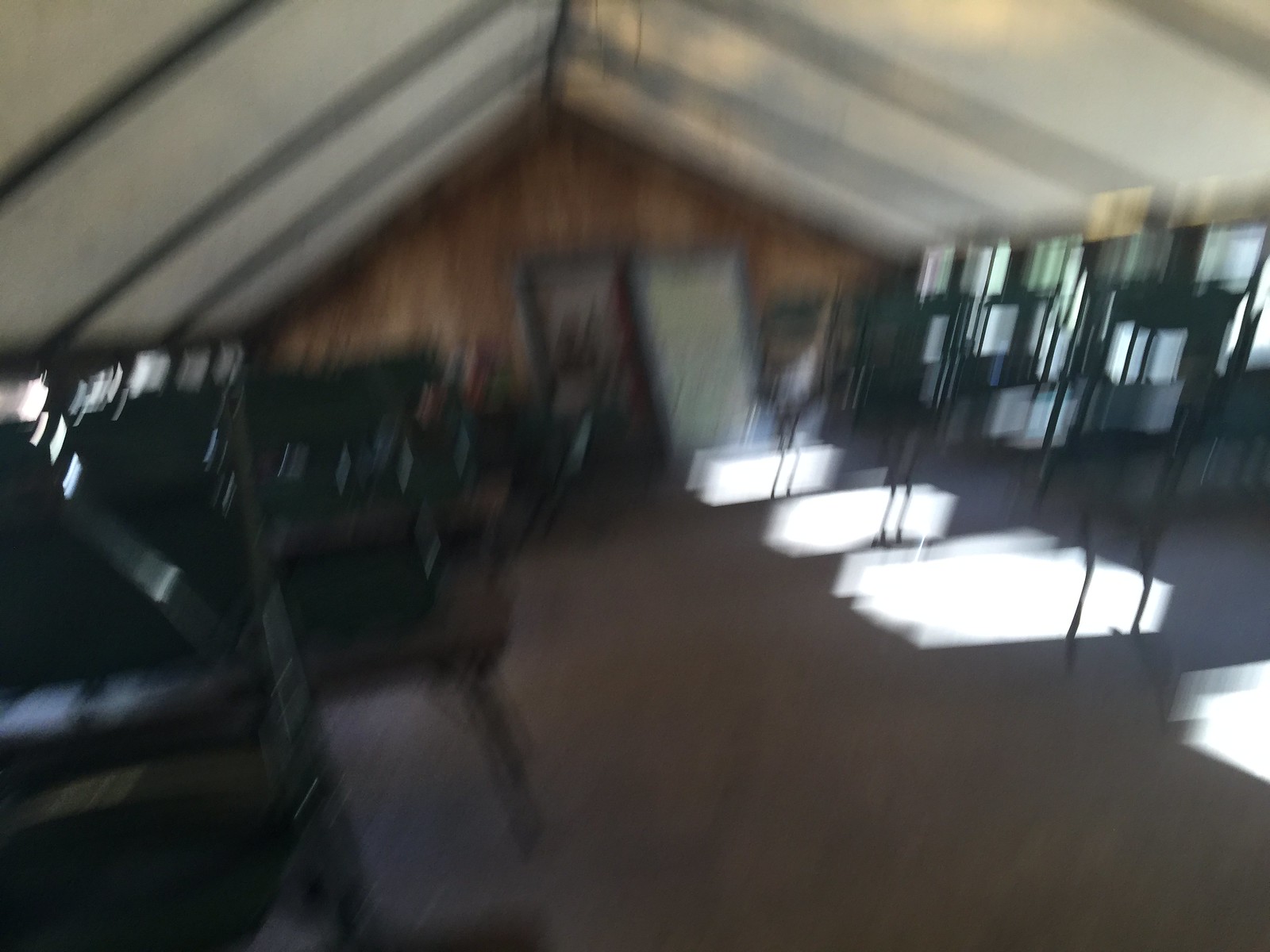A blurry photograph captures the interior of a room with brown walls and floors, taken from an angle that looks across the space. The room features several green chairs scattered around. Four distinct patches of sunlight, likely streaming through windows, illuminate the floor along the length of the wall. Large frames, possibly pictures or mirrors, rest against the back wall. The ceiling is white and has a vaulted shape, forming an inverted V that rises from the left side, peaks in the middle, and descends to the right.